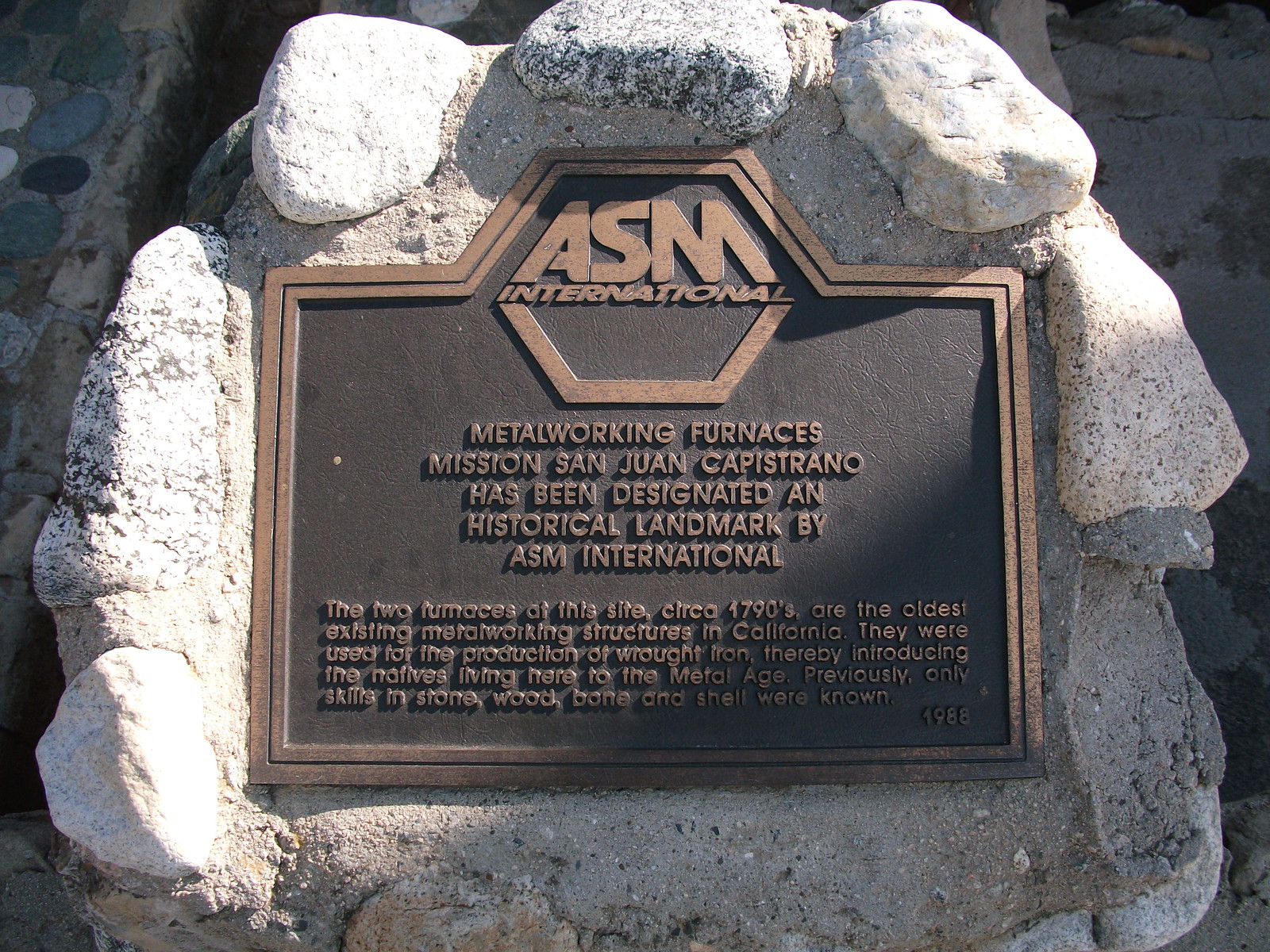The image depicts a bronze plaque embedded in a cement circle, surrounded by a series of large rocks forming a circular border. The plaque itself features a dark brown inner area with light brown raised bronze lettering. At the very top in large, bold letters, it reads "ASM International." Below this, in smaller letters, the plaque states: "Metal Working Furnaces Mission San Juan Capistrano has been designated a historical landmark by ASM International." The text further elaborates that the two furnaces at this site, dating back to the 1790s, are the oldest existing metalwork structures in California. They were used for the production of wrought iron, thereby introducing the indigenous inhabitants to the metal age. The plaque is positioned horizontally, facing upwards, making it easy for viewers to look down and read the historical information.